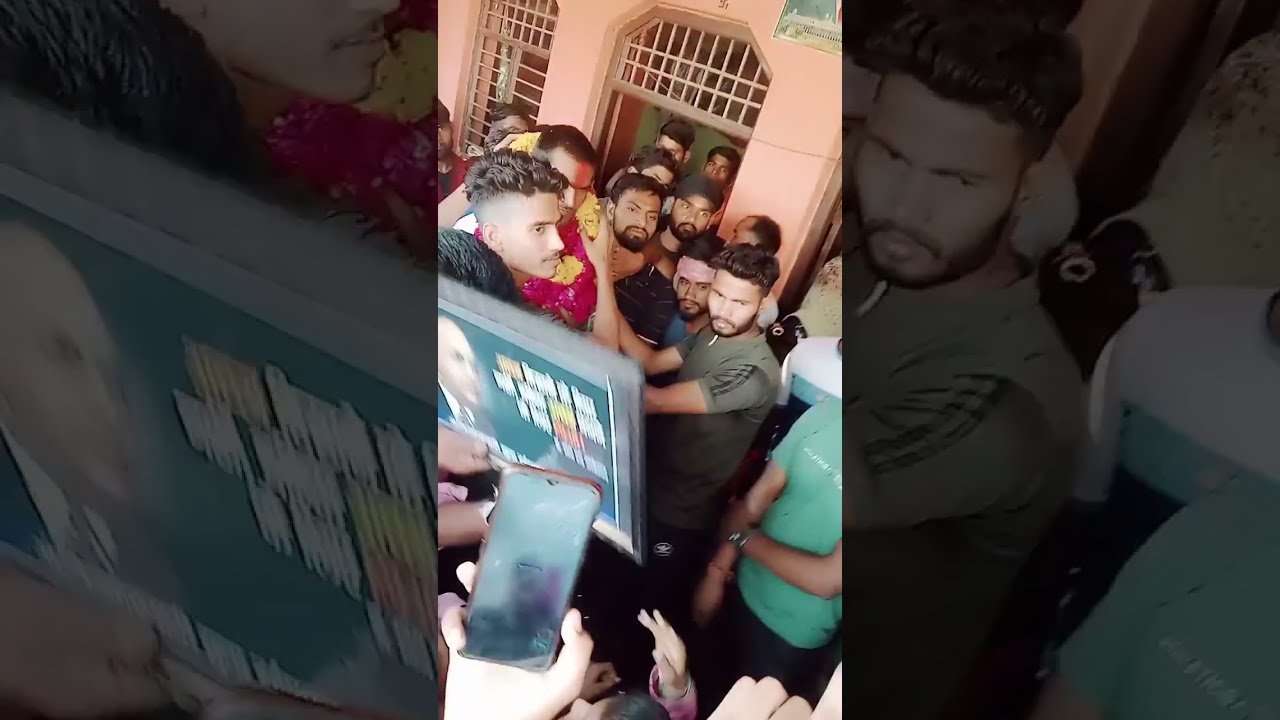The image is a rectangular composite broken into three panels, with the center panel brightly lit and the left and right panels darkened. The central panel features a man adorned with several pink and yellow leis around his neck, standing amidst a crowd. The crowd includes various men and women, some in short-sleeved polo shirts of blue, orange, and black. Behind the crowd is a salmon-colored building with barred windows and a gated doorway, where two people are standing. The left panel is a close-up of a man in a blue checkered shirt, showing the back of his head and another man's profile. The right panel captures part of the same scene with three men in dark shirts, one of whom is facing away from the viewer. The repeated side panels give a zoomed-in perspective of the central image, emphasizing the gathering and its setting.